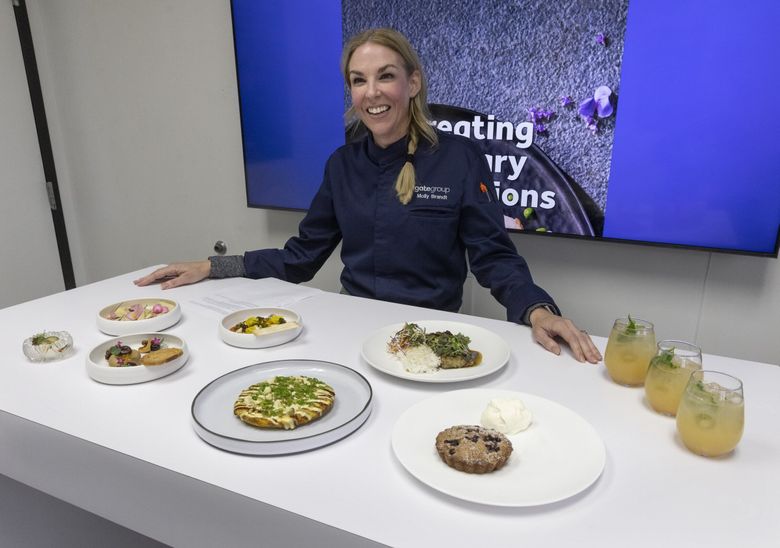In the image, a woman with blonde hair tied in a ponytail draped over her left shoulder is smiling and looking slightly to her left. She is wearing a long-sleeved blue sweater with white text that reads "Gate Group" on the left side of her chest, possibly accompanied by her name, but it is too small to discern. Seated at a white rectangular table angled towards the lower right, the table is adorned with various white plates. There are larger plates on the right and smaller ones on the left, each artistically displaying a variety of desserts, including cookies with green and yellow toppings. The plate nearest to her appears to contain something white, possibly rice. To her left, there are three cups containing a yellowish drink with ice cubes and a lime garnish. Behind her is a TV screen displaying a blue backdrop with some kind of slideshow in the middle. The background wall is white, complementing the overall clean and organized setting.